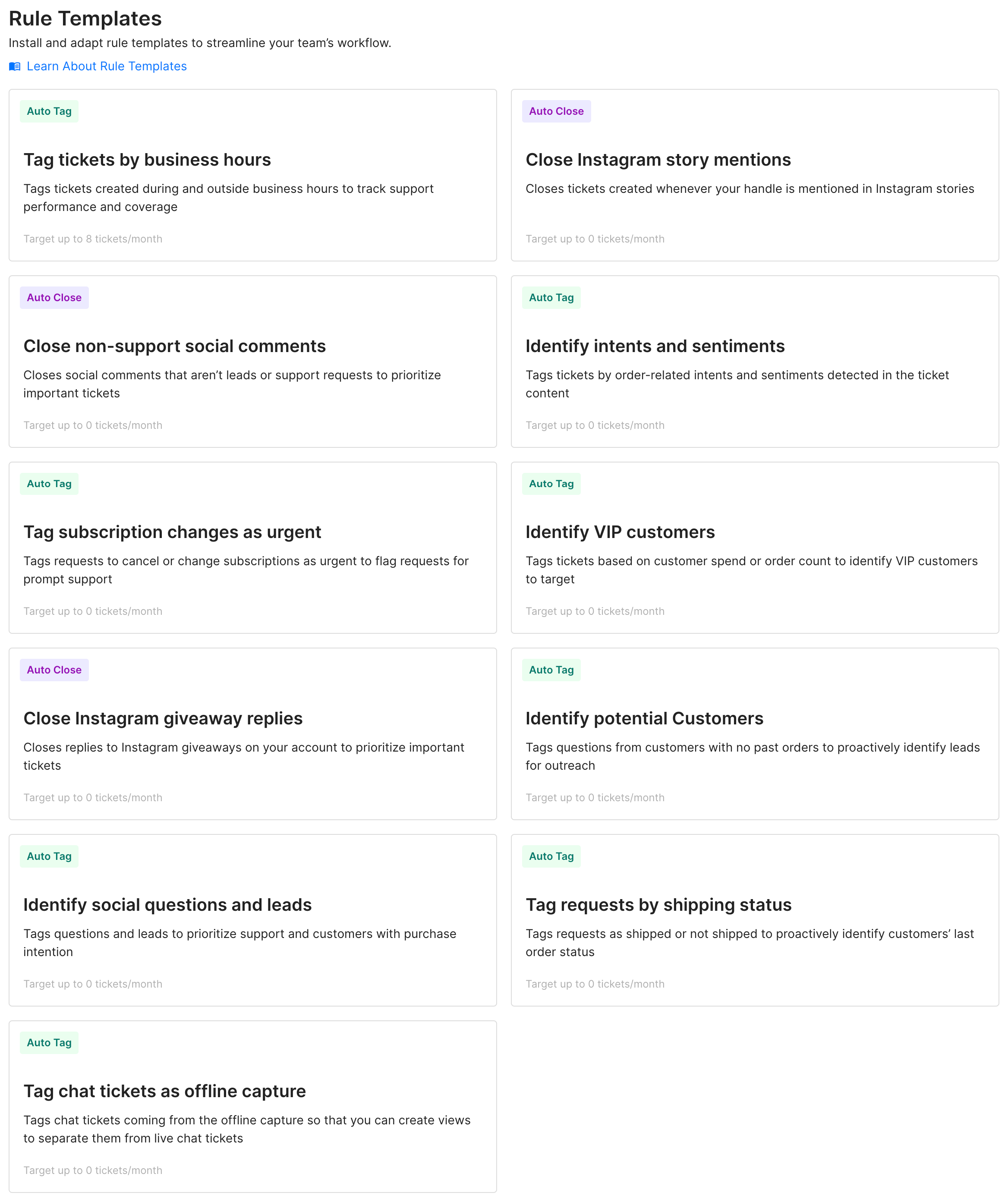The image captures a screenshot from a website, featuring a section titled "Rule Templates." This title is prominently displayed in black text with both "R" and "T" capitalized. Directly beneath it, a smaller subheading reads, "Install and adapt rule templates to streamline your team's workflow." Further down, a blue hyperlink invites users to "Learn about rule templates."

The main body of the screenshot is divided into two rows of rectangular boxes, each representing different rule templates with a distinct color coding. 

In the first row:
1. A light green rectangle titled "Auto Tag" details a rule in which tickets are tagged by business hours.
2. A pale purple rectangle titled "Auto Close" describes a rule for closing non-support social comments.
3. Another light green rectangle, also titled "Auto Tag," specifies a rule for tagging subscription changes as urgent.
4. A pale purple rectangle titled "Auto Close" specifies a rule for closing Instagram giveaway replies.

In the second row:
1. A light green rectangle labeled "Identify Social Questions and Leads."
2. Another light green rectangle informing "Tag Chat Tickets as Offline Capture."
3. A pale purple rectangle titled "Close Instagram Story Mentions."
4. A series of four light green rectangles describing:
   - "Identify Intents and Sentiments."
   - "Identify VIP Customers."
   - "Identify Potential Customers."
   - "Tag Requests by Shipping Status."

Each rectangle encompasses a succinct description of the rule it represents, effectively providing an organized and visually distinct layout for users to understand and utilize various rule templates.